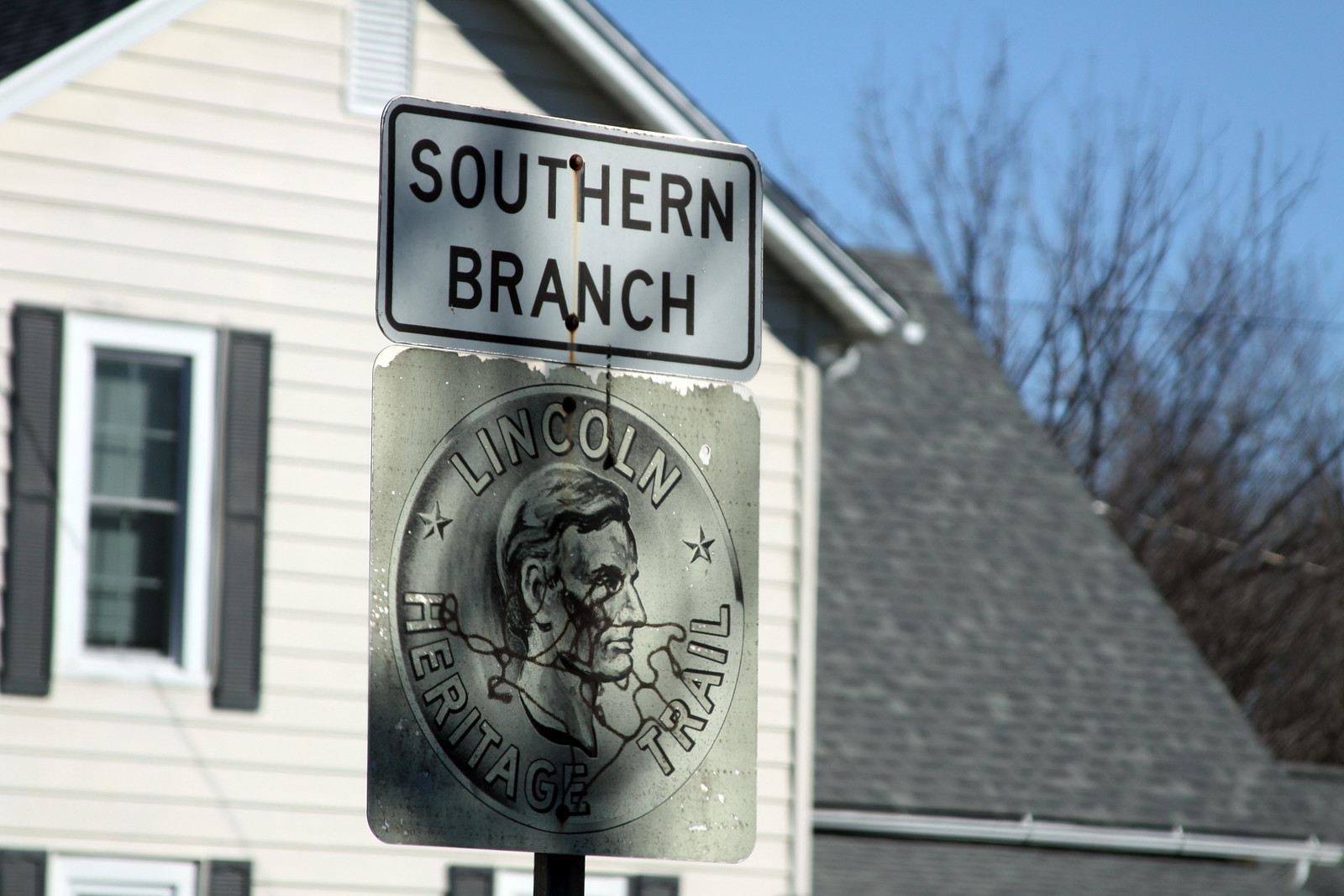This is an outdoor image capturing a historical marker for the Lincoln Heritage Trail, prominently featured in the center. The sign comprises a white rectangular plaque at the top that reads "Southern Branch" in black text with a black border. Below it is a gray, weathered sign designed to resemble a penny, featuring the profile of Abraham Lincoln with the text "Lincoln Heritage Trail" encircling his face. A trail map line runs across the bust, and two stars frame the design. The marker is mounted on a pole located in a residential neighborhood. The background showcases a large beige house with white siding, black-trimmed windows, white gutters, a black composition roofline, and dark green shutters. The scene is set in what appears to be winter, as a nearby tree is nearly bare, and the blue sky suggests it is daytime, likely late afternoon. Additional elements include power lines and trees situated further behind the house.